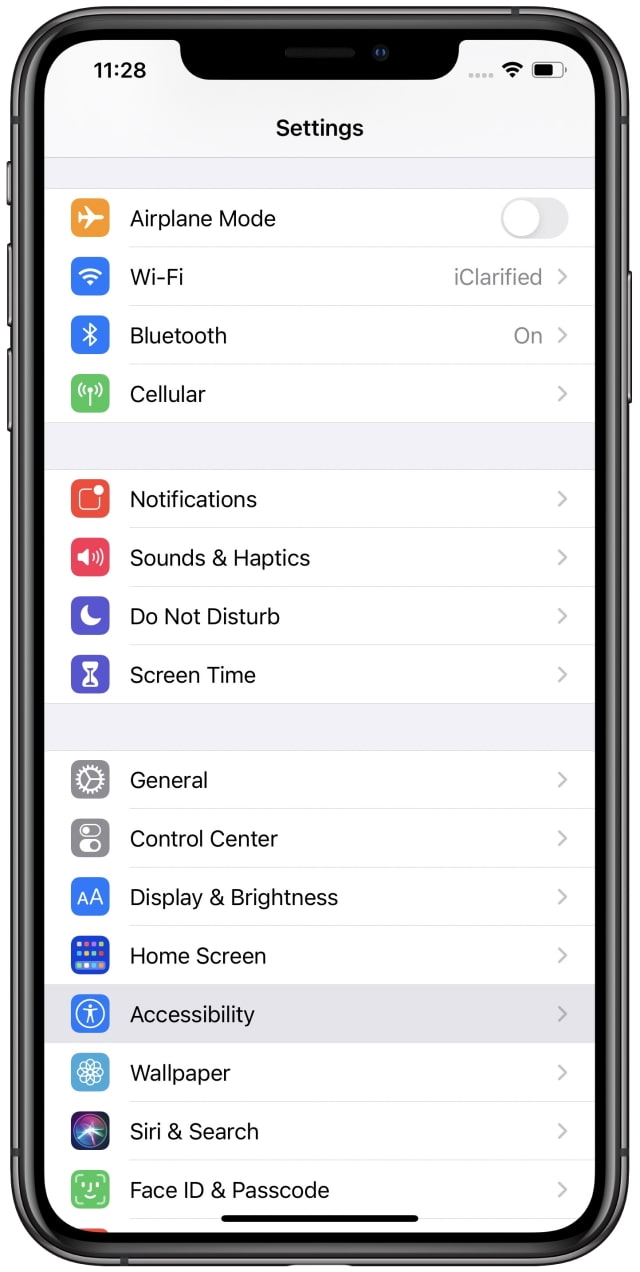This vertical image appears to be a photograph of someone's smartphone screen. The phone itself, enclosed within a black rim, is visible in the image. At the top left-hand corner, the time is displayed as 11:28. On the top right-hand corner, there are the three vertical dots indicating more options, the Wi-Fi icon, and the battery icon.

The screen shows the 'Settings' menu. Starting from the top, icons and their corresponding labels are arranged in a list format. The first item is 'Airplane Mode,' which is toggled off. Below that, we see 'Wi-Fi' (enabled), 'Bluetooth' (on), and 'Cellular.' 

The next section of the settings menu includes 'Notifications,' 'Sounds & Haptics,' 'Do Not Disturb,' and 'Screen Time.' 

In the final section visible, items listed include 'General,' 'Control Center,' 'Display & Brightness,' 'Home Screen,' and 'Accessibility' (highlighted), followed by 'Wallpaper,' 'Siri & Search,' and 'Face ID & Passcode.'